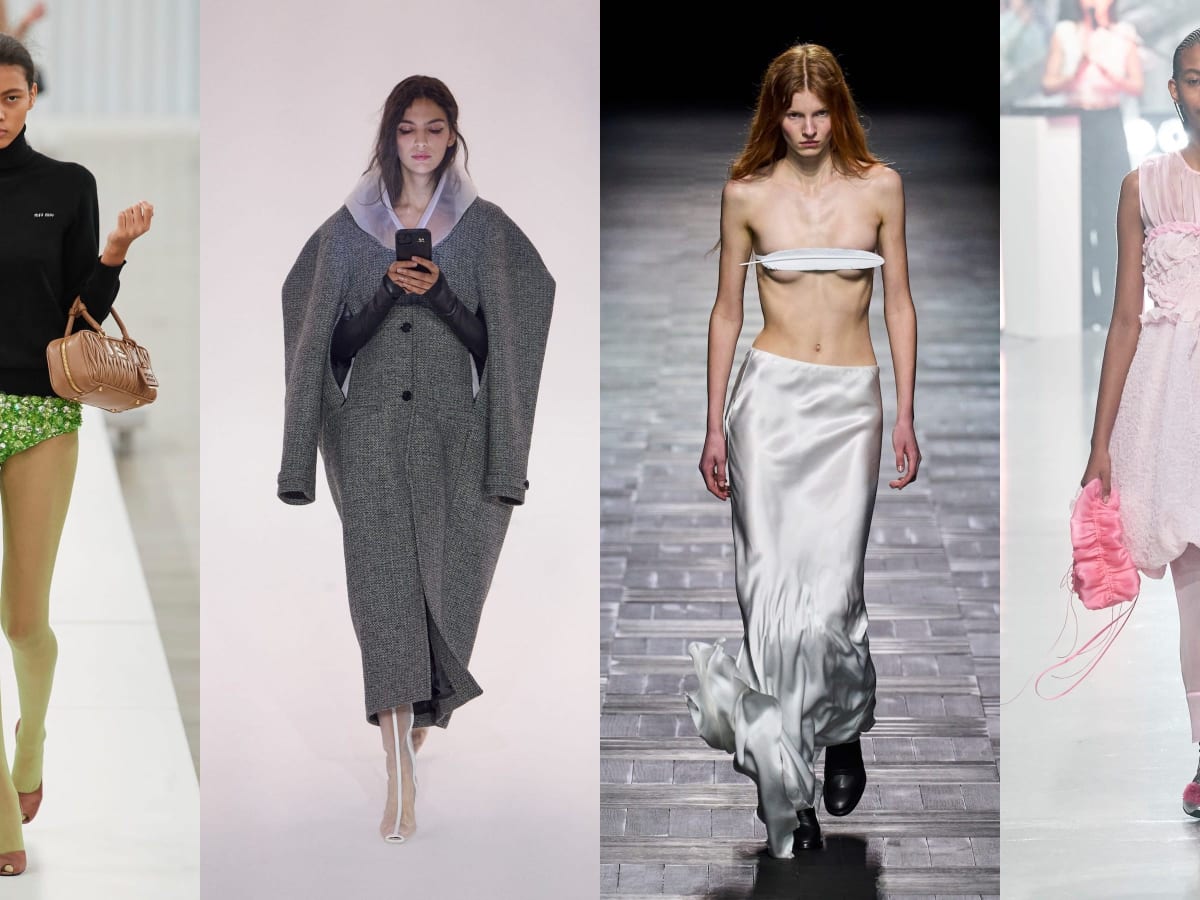This series of four narrow, vertical photographs showcases high fashion models walking down the runway. The images on the far left and far right are cropped, showing only half of the models.

The first image, on the far left, features a dark-skinned model with sleek, pulled-back hair. She is dressed in a black turtleneck sweater, green floral panties, and cream-colored leggings. Completing her look, she wears pink open-toe high heels and carries a small tan handbag. Her poised stance and raised arm holding the bag suggest a confident stride.

The second image depicts a brown-haired model with olive skin donning a distinctive gray coat that combines elements of a cape and sleeved coat, although her arms emerge through slits rather than the sleeves. She holds a cell phone and gazes down at it. Her ensemble is rounded out with sheer, high-top white boots, highlighting a blend of modern and classic styles.

In the third image, we see a very skinny model with striking red hair cascading down. She wears a strip of white cloth covering her breasts, paired with a long, shiny white skirt that glides over the gray tiled runway floor. Her outfit is accessorized with black shoes, creating a contrast with the light tones of her attire.

The final image on the far right shows half of a model with dark skin and dark hair, dressed in a light pink, knee-length skirt that appears frilly and fashionable. She carries a pink fabric purse in her right hand, adding to her chic, monochromatic ensemble.

Overall, each photograph captures the unique style and poise of the models, highlighting diverse fashion elements and accessories as they confidently grace the runway.